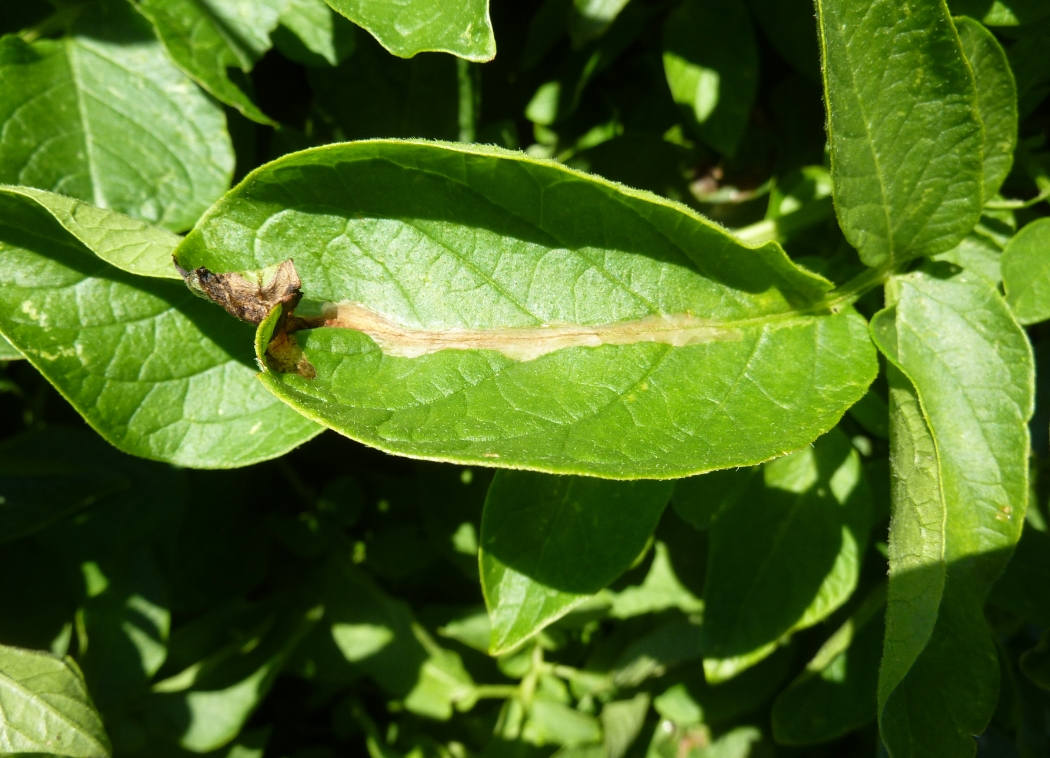This close-up photograph captures a green oval leaf under attack by the invasive potato tuber moth, a pest prevalent in both Indonesia and Western Australia. The potato tuber moth is characterized by its long brown body adorned with dark flecks on its wings. The edge of the leaf appears curled and the central vein has turned brown, indicating the leaf is nearing death. Within the scene, the egg stage of the moth is visible, having hatched into larvae. A noticeable cocoon encloses a brown larva, poised to emerge and continue feasting on the lush potato leaves, which occupy the background as well.